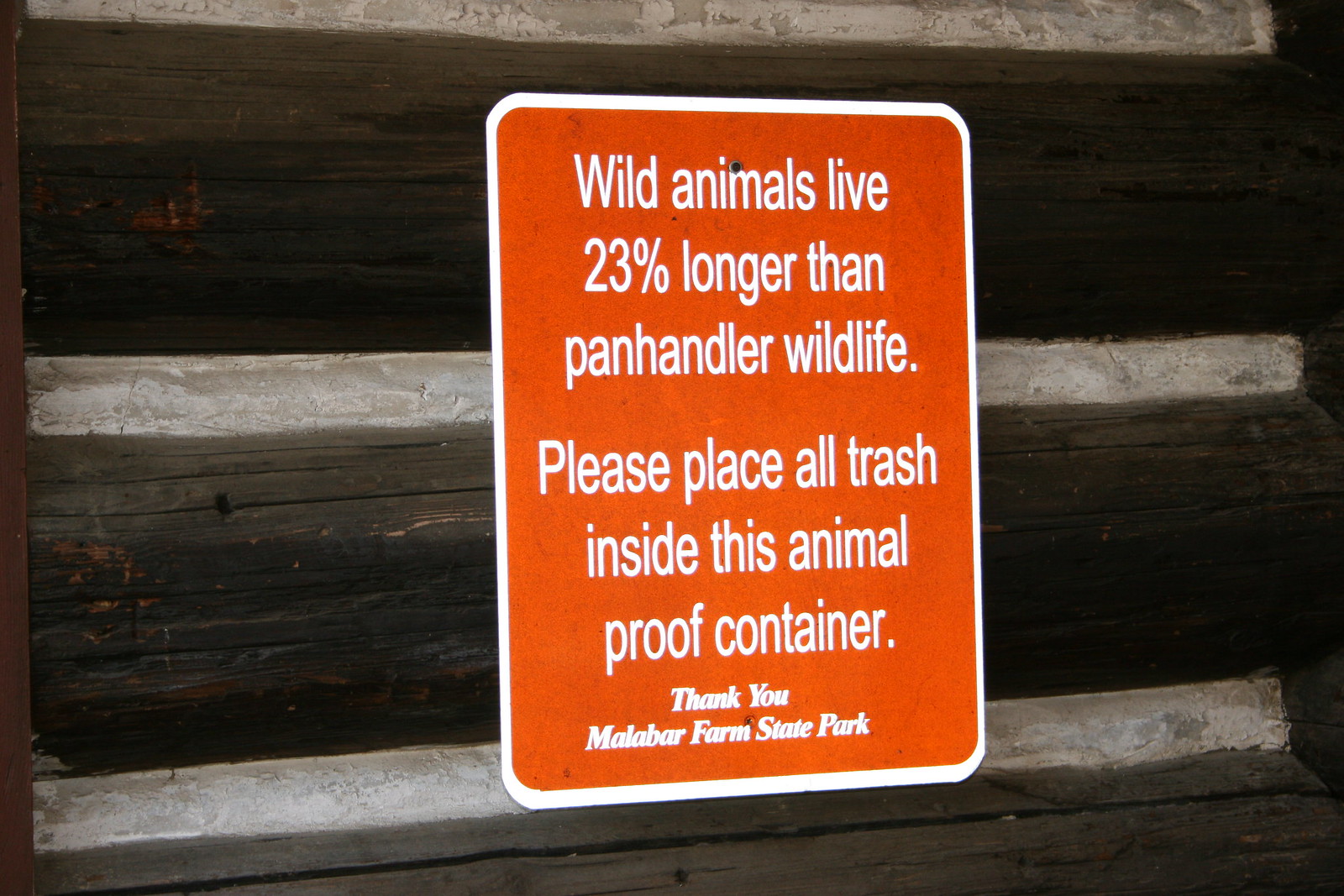The image shows a close-up of an orange, possibly thin metal sign with a white border and white text, affixed to a wooden structure comprised of three visible beams. The sign, located at Malabar Farm State Park, features different fonts for emphasis: the main message, "Wild animals live 23% longer than panhandler wildlife. Please place all trash inside this animal-proof container. Thank you," is in Arial Narrow font, while "Malabar Farm State Park" is in white italics with a cursive style. The sign is designed to inform visitors to properly dispose of their trash in designated containers to prevent wildlife from becoming dependent on human food, thereby supporting healthier, more natural behaviors among the animals. The wooden structure the sign is mounted on appears to be at a slight angle, suggesting it could be part of a larger outdoor installation aimed at protecting the park's ecosystem.